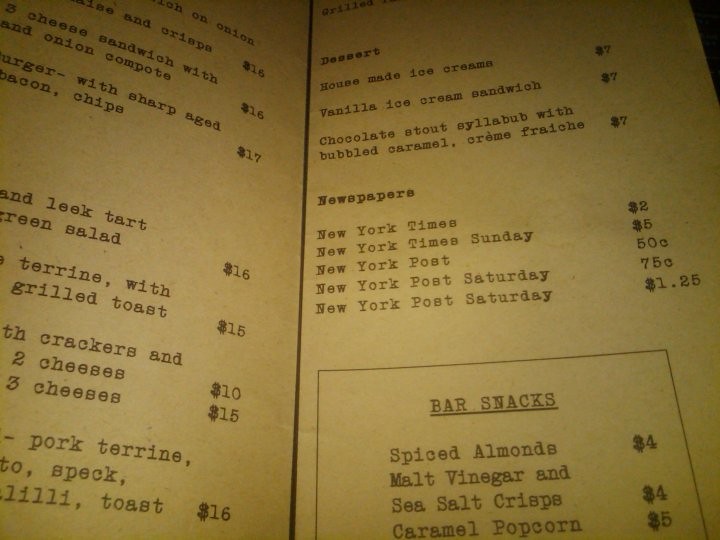A photograph of a thick white menu with black specks and grainy quality. The menu is printed on a single sheet of white stock paper with black text. The left side features a partially visible list of food items, with prices ranging from $10 to $17. On the right side, the section titles and item details are much clearer. It lists "Dessert" options in black font: Housemade Ice Cream ($7), Vanilla Ice Cream Sandwich ($7), and Chocolate Stout Syllabub with Bubble Caramel Crème Fraîche ($7).

Below the dessert options, there's a list of "Newspapers" with pricing: The New York Times ($2), The New York Times Sunday edition ($5), New York Post ($0.50), New York Post Saturday ($0.75), and another price for New York Post Saturday ($1.25).

The lower section of the menu denotes "Bar Snacks," including Spiced Almonds ($4), Malt Vinegar and Sea Salt Crisp ($4), and Caramel Popcorn ($5).